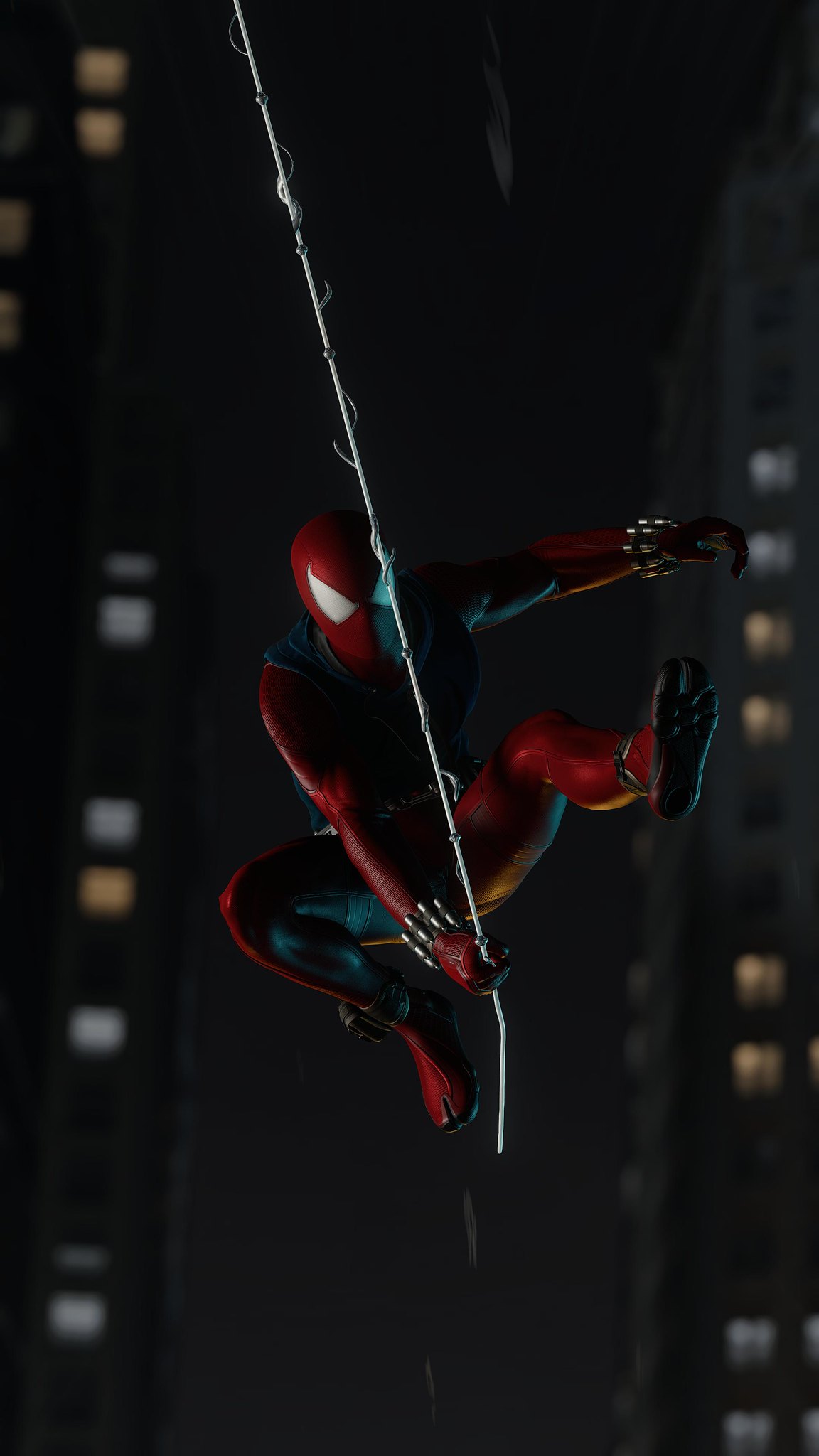The photograph showcases a striking, computer-generated image of Spider-Man set against a predominantly black background reminiscent of a nighttime cityscape. The scene is framed in a portrait orientation, several times taller than it is wide, with two towering skyscrapers flanking the left and right edges of the frame. Some windows in these skyscrapers are illuminated, piercing the darkness with rectangular pools of light.

At the forefront of the image, Spider-Man, donned in his classic costume - a red and blue spandex suit with large white triangle-shaped eyes on his mask, skillfully manipulates a thin, silvery cable. The cable, resembling a web, stretches diagonally from his grip, up and out of the top of the image, wrapping around itself for support. Spider-Man is captured in an acrobatic pose, reminiscent of a baseball catcher’s crouch but with dynamic twists: his right arm extends downwards to grasp the cable below his waist, while his left arm stretches outward horizontally to the right, fingers curling towards the ground.

His red and black wristbands, seemingly equipped with web-producing gadgets, add a technological flair to his ensemble, which also includes detailed, sturdy boots. Spider-Man's right leg is bent close to his body, and his left leg kicks forward, allowing the viewer a glimpse of the sole of his foot, as he appears mid-leap or climb. The dramatic lighting and careful composition highlight Spider-Man’s agile form and his preparedness to swing effortlessly through the urban landscape.